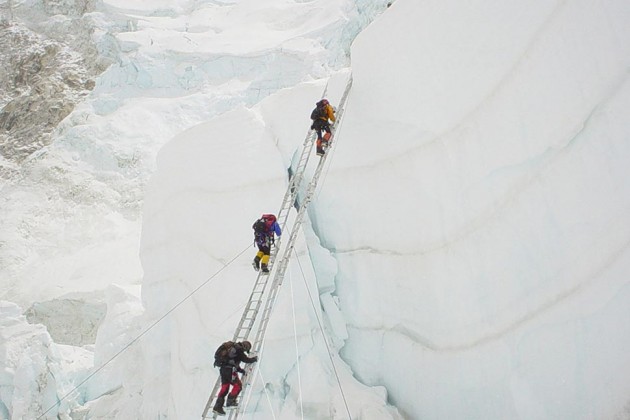The photograph captures an intense outdoor winter adventure scene, where three climbers are ascending a massive, grey ladder that's propped against what appears to be a snow-covered mountain or a large snow structure, possibly resembling a hill or avalanche of snow. 

The ladder is lengthy, extending to impressive heights, marked with multiple rungs and supported by safety cables. At the top of the ladder, a climber dressed in a red outfit is cautiously making their way up. Midway up, another climber can be seen sporting a blue and yellow outfit. At the very bottom, the third climber is in a blue and red outfit. All climbers are equipped with backpacks and are bundled up in heavy winter gear, including hats, to protect against the harsh, snowy environment. The background is dominated by the white, snowy texture, reinforcing the wintry and adventurous nature of the setting.